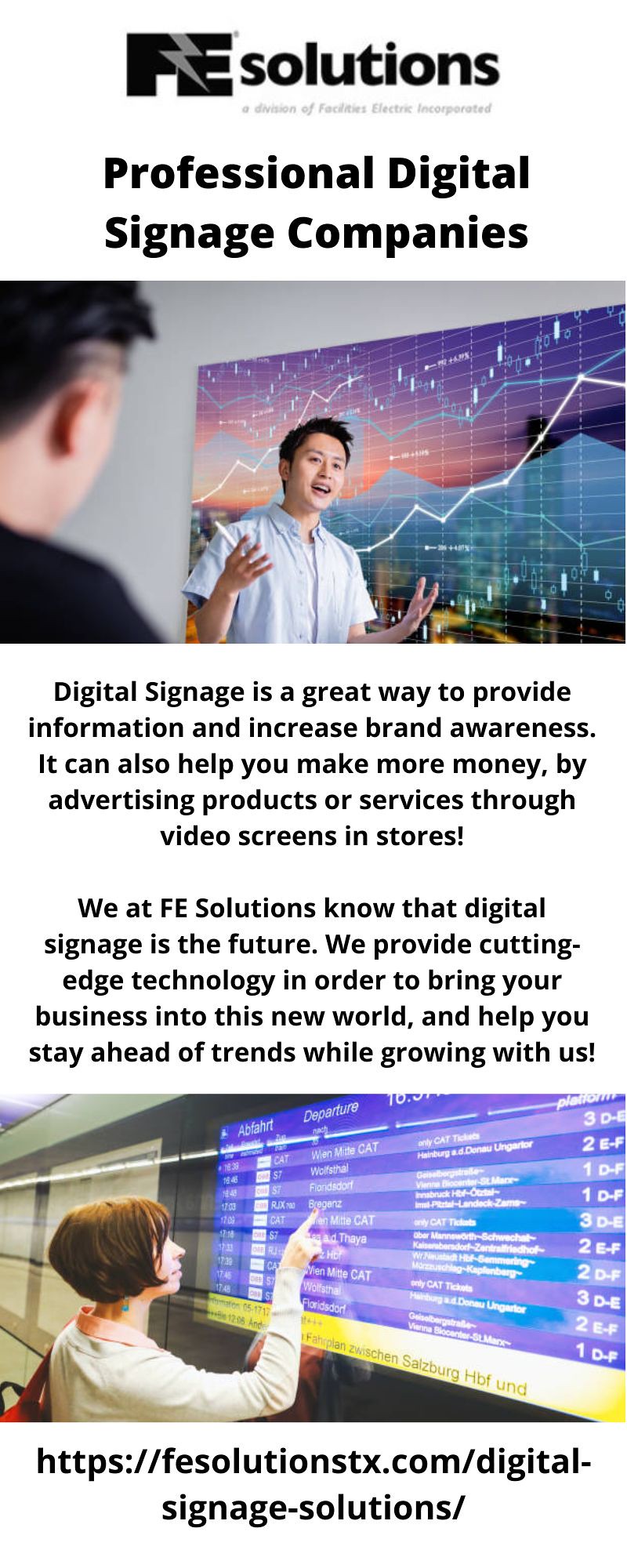This digital ad for FE Solutions, displayed in a vertical column on a white background, prominently features a bold black header reading "FE Solutions." Below that, a subheading in slightly italicized black sans-serif font states, "Professional Digital Signage Companies." The ad is visually divided into sections with images and text.

The first section displays an image of a young Asian male in a short-sleeve button-down shirt, standing in front of a colorful graph. He holds a marker in his upraised right hand. To his left, a second Asian male is partially visible from the back, wearing a black shirt and appearing to observe the first man.

Beneath this image, a centered paragraph in black text reads: "Digital signage is a great way to provide information and increase brand awareness. It can also help you make more money by advertising products or services through video screens in stores!"

A subsequent paragraph states: "We at FE Solutions know that digital signage is the future. We provide cutting-edge technology to bring your business into this new world and help you stay ahead of trends while growing with us!"

Following the text, a second image features a young woman with a dark pageboy haircut, wearing a white long-sleeve sweater. She stands left in profile, her raised right arm pointing to a large blue and purple sign with several lines of unreadable white text.

The ad concludes with the website, displayed in small lowercase black text: "https://fesolutionstx.com/digital-signage-solutions/"